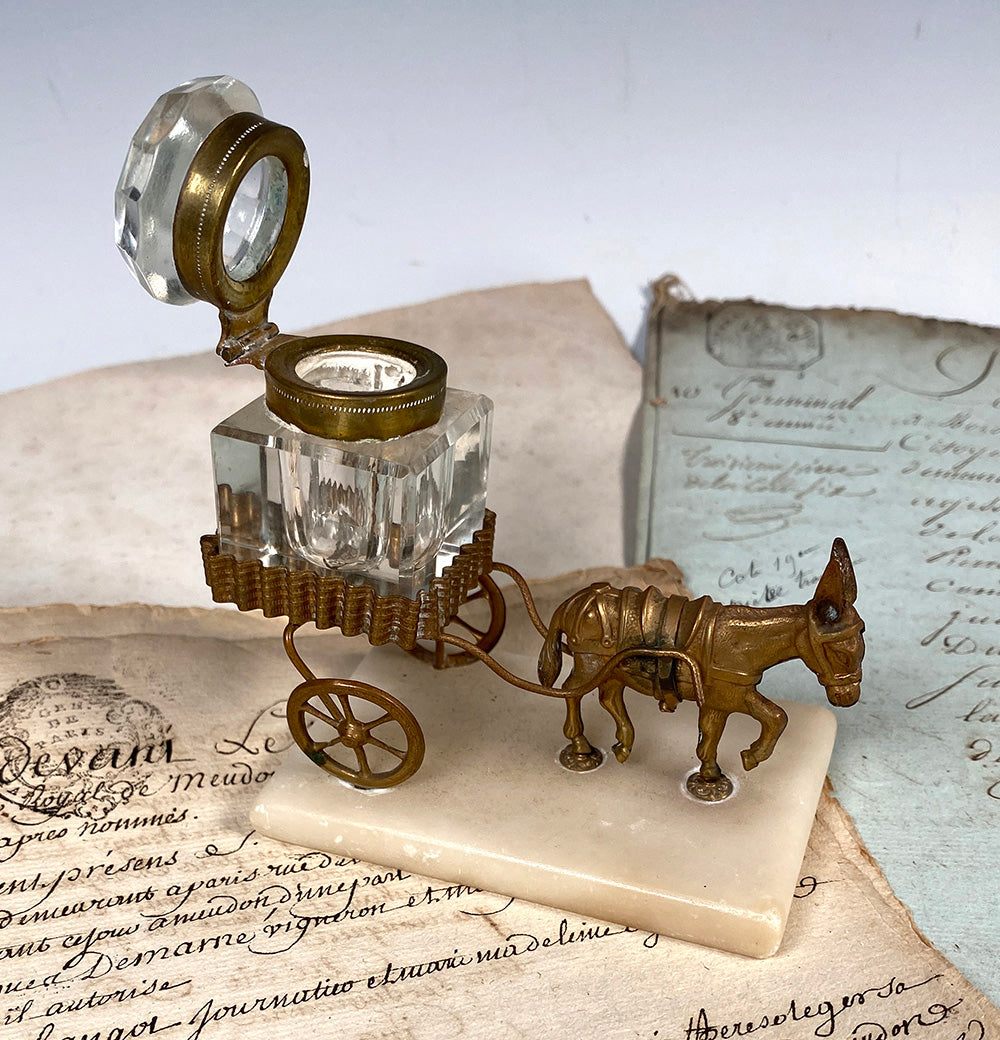The image portrays a detailed still life composition set against a light blue and whiteish-gray background. At the center, there is an intricate brass figurine of a donkey pulling a two-wheeled cart, which is mounted on a slab of white marble. The cart holds a small, open crystal container identified as an inkwell, topped with a brass and additional crystal lid. Surrounding the marble base are pieces of aged handwritten parchment paper, featuring calligraphy and possibly Latin or Spanish text. This layered arrangement of materials and textures, from the brass and crystal to the parchment and marble, creates a rich tableau that juxtaposes elements of age and artistry.